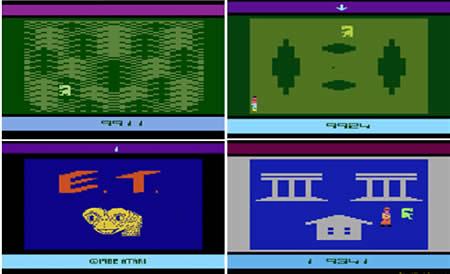This image showcases four vintage video game screenshots, each displaying distinct graphics and elements. 

1. **Top Left**: The first screenshot predominantly features various types of trees—light green and dark green—set against a grassy background. Among the trees stands a small, yellow creature reminiscent of E.T. The screen also has a blue strip at the bottom with the number "9911" and a purple strip across the top.

2. **Top Right**: This image displays a game with a purple strip along the top and a lighter blue strip at the bottom, featuring the number "9924". Noteworthy are the two vertically aligned ovals on either side and two horizontally aligned ovals in the middle. At the top of the screen is the E.T. creature, while at the bottom is a small human figure.

3. **Bottom Left**: The third image prominently features the text "Pipe Atari" and "E.T." in orange letters, along with an illustration of E.T. the Extra-Terrestrial.

4. **Bottom Right**: In the final screenshot, two gray structures—possibly buildings—are visible at the bottom. Above, the scene includes what appear to be two bridges, along with a human figure and the E.T. creature, accompanied by the number "9341".

These images evoke the nostalgic aesthetics of early video games, characterized by their simple yet iconic graphics and characters.